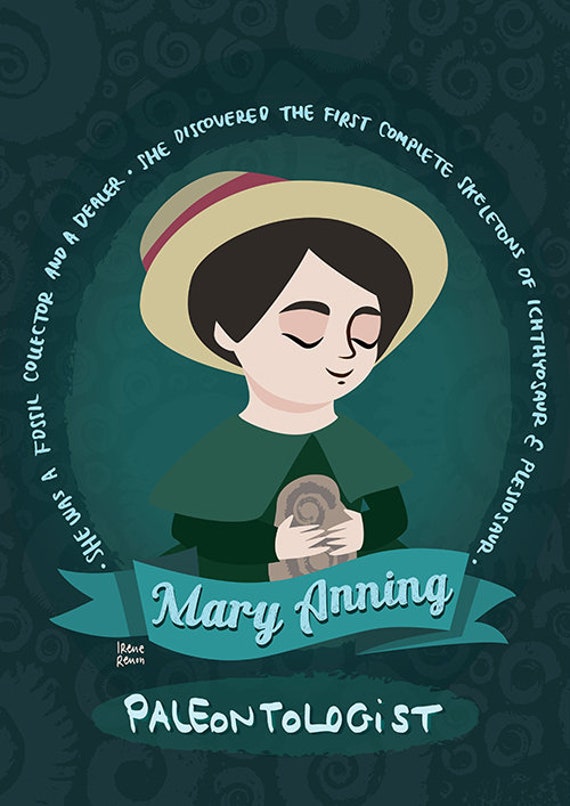This detailed illustration honors Mary Anning, framed by a dark green background adorned with subtle, swirly circles. At the center, against a lighter green backdrop, is a simplified, cartoon-like image of Mary Anning herself. She sports a tan straw hat with a red ribbon, her brown hair stylishly parted to the side. With her eyes gently closed and a soft smile, she clutches a tan, fossil-like object in her hands. Mary is dressed in a green dress, complemented by a light-green shawl. Encircling her portrait is a caption noting her significant achievements, stating she was a fossil collector and dealer who discovered the first complete skeletons of Ichthyosaur and Plesiosaur. Below her image, a teal ribbon reads "Mary Anning," with "paleontologist" written underneath. The artist's signature, "Irene Rehmen," is also included, honoring her contribution to this tribute.